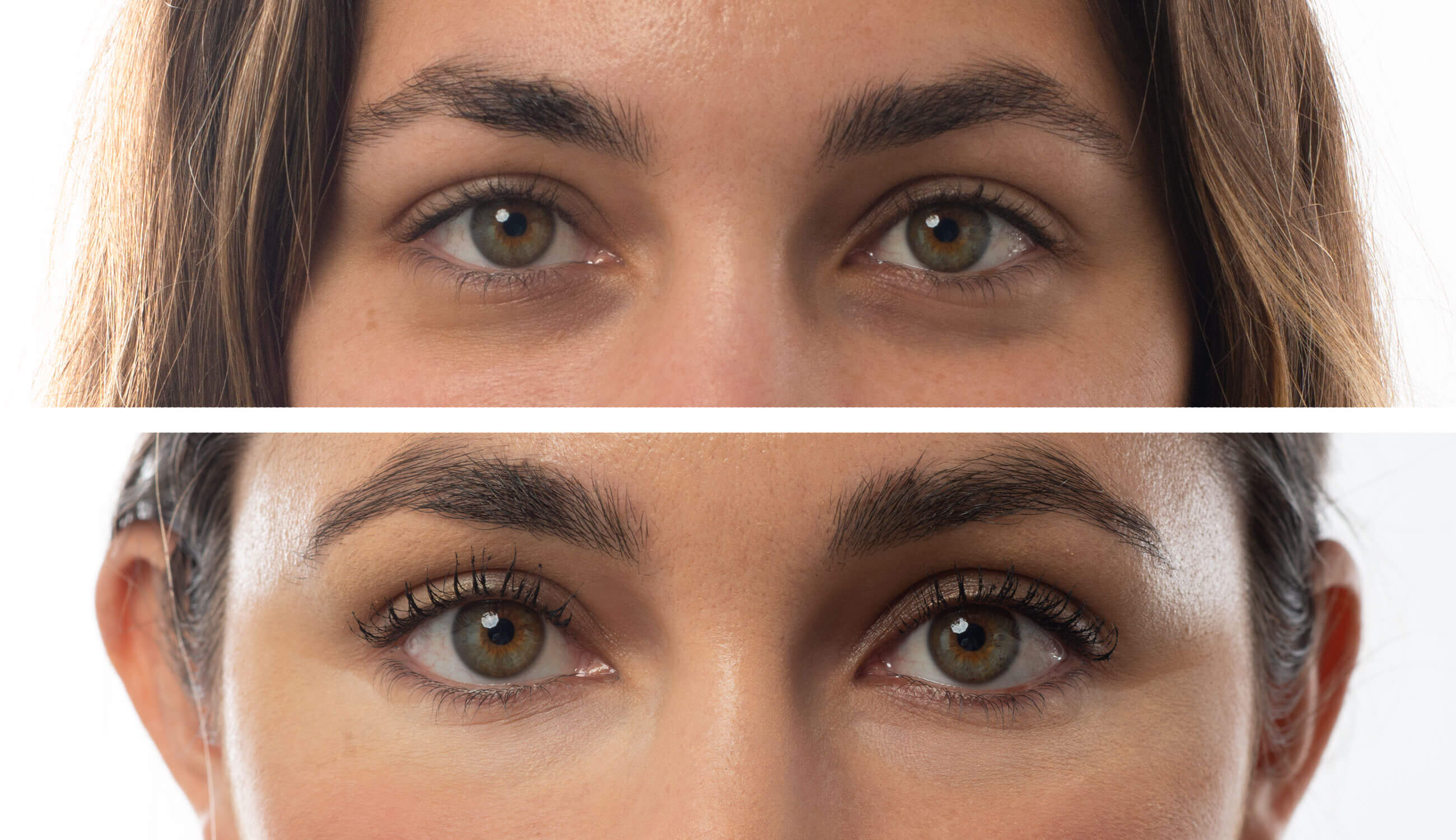This split image consists of two closely cropped, rectangular photographs, one positioned above the other, with a small horizontal white line dividing them. Both images focus on the face of a woman from just above her eyebrows to the top of her nose, emphasizing her eyes and surrounding features. In the top image, the woman has straight brown hair framing her face, brownish-green eyes, and dark brown eyebrows that peak in the center. She is not wearing makeup, presenting a natural and real look that accentuates her beauty. In the bottom image, the same woman appears with her hair pulled back, showcasing her ears. Her eyes remain the same captivating hue, but she now has longer eyelashes coated with slightly clumpy mascara, along with eyeliner and foundation, presenting a more polished appearance. Despite the addition of makeup, her eyebrows remain the same, and her overall look is subtly enhanced while maintaining her inherent beauty.